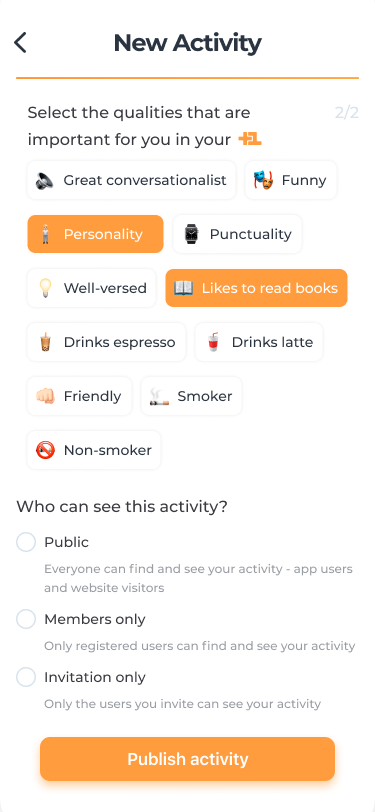This image features a mobile device screenshot, displaying a page from an app or website with a clean, white background. At the top, there is a left-pointing arrow icon and a bold black banner reading "New Activity". Directly below this header is an orange line, followed by the instruction to "Select the qualities that are important in your...". Next to this instruction, there is an icon that appears to resemble a plus sign overlaying a store or building icon.

Beneath this, the text "2 of 2" indicates the second page or section of the activity. The screen presents a list of qualities with the heading "Select the qualities that are important in your...". The qualities listed are: "Great conversationalist", "Funny", "Personality", "Punctuality", "Well-versed", "Likes to read books", "Drinks espresso", "Drinks latte", "Friendly", and "Smoker or non-smoker". The user selections of "Personality" and "Likes to read books" are highlighted in orange, indicating these choices have been selected.

Following the list, the text "Who can see this activity?" is presented, with three visibility options below:
1. "Public" - where everyone, including app and website users, can find and see the activity.
2. "Members only" - where only registered users have access to view the activity.
3. "Invitation only" - where only invited users can see the activity.

At the bottom of the screen, an orange button labeled "Publish Activity" is prominently displayed, inviting the user to finalize and share their activity preferences.